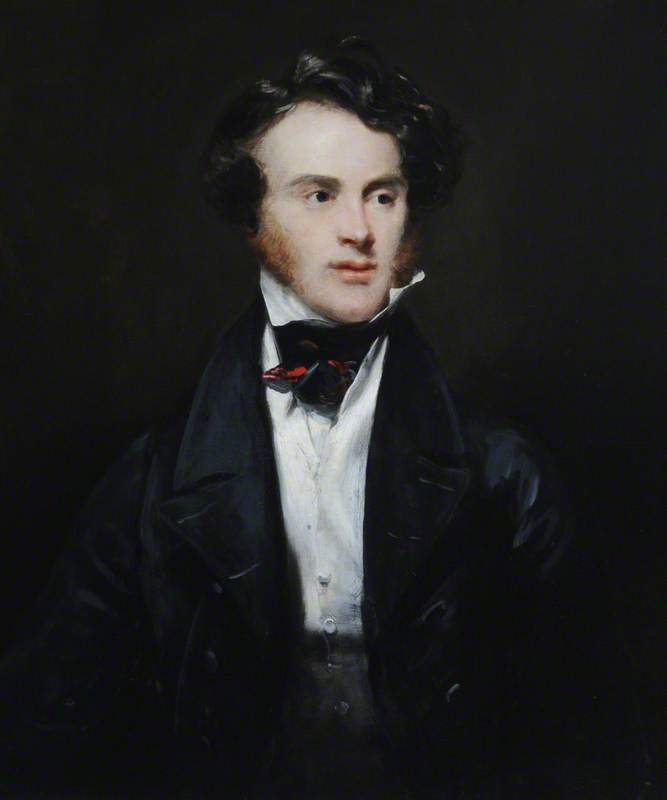This image depicts a hand-painted portrait of a man from the 1800s, positioned against a stark, dark background that emphasizes the solemn tone of the painting. His face is pale with a clean-shaven chin, exhibiting wavy dark brown hair and distinct long sideburns that appear lighter, almost orange-brown in hue. He gazes slightly to the right, adding a contemplative demeanor to his visage. Dressed in old-fashioned attire, he wears a sizable, thick black coat over a crisp white button-down shirt. Underneath his collar, he sports a necktie with hints of green and red, partially stuffed inside his shirt. The overall ambiance of the painting is somber and reflective, with no additional elements in the dark background to distract from the solitary figure of the man.